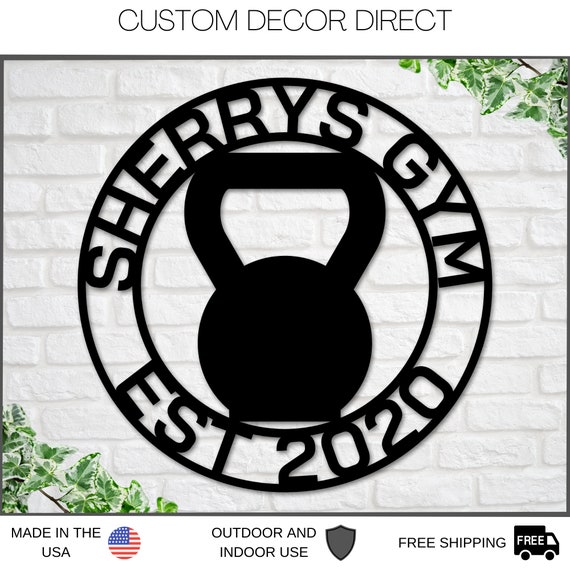The image is an advertising logo for "Sherry's Gym," established in 2020, created by Custom Decor Direct. It features a central black kettlebell encircled by two rings, with the gym's name displayed between the circular lines. The background is a white brick wall with greenery in the top right and bottom left corners. Below the main image, there are multiple badges: "Made in the USA" with an American flag, "Outdoor and Indoor Use" with a shield, and "Free Shipping" with a box truck and the word "FREE." This suggests the sign is available for order and customization, suitable for both indoor and outdoor settings while emphasizing its domestic manufacture and free shipping offer.